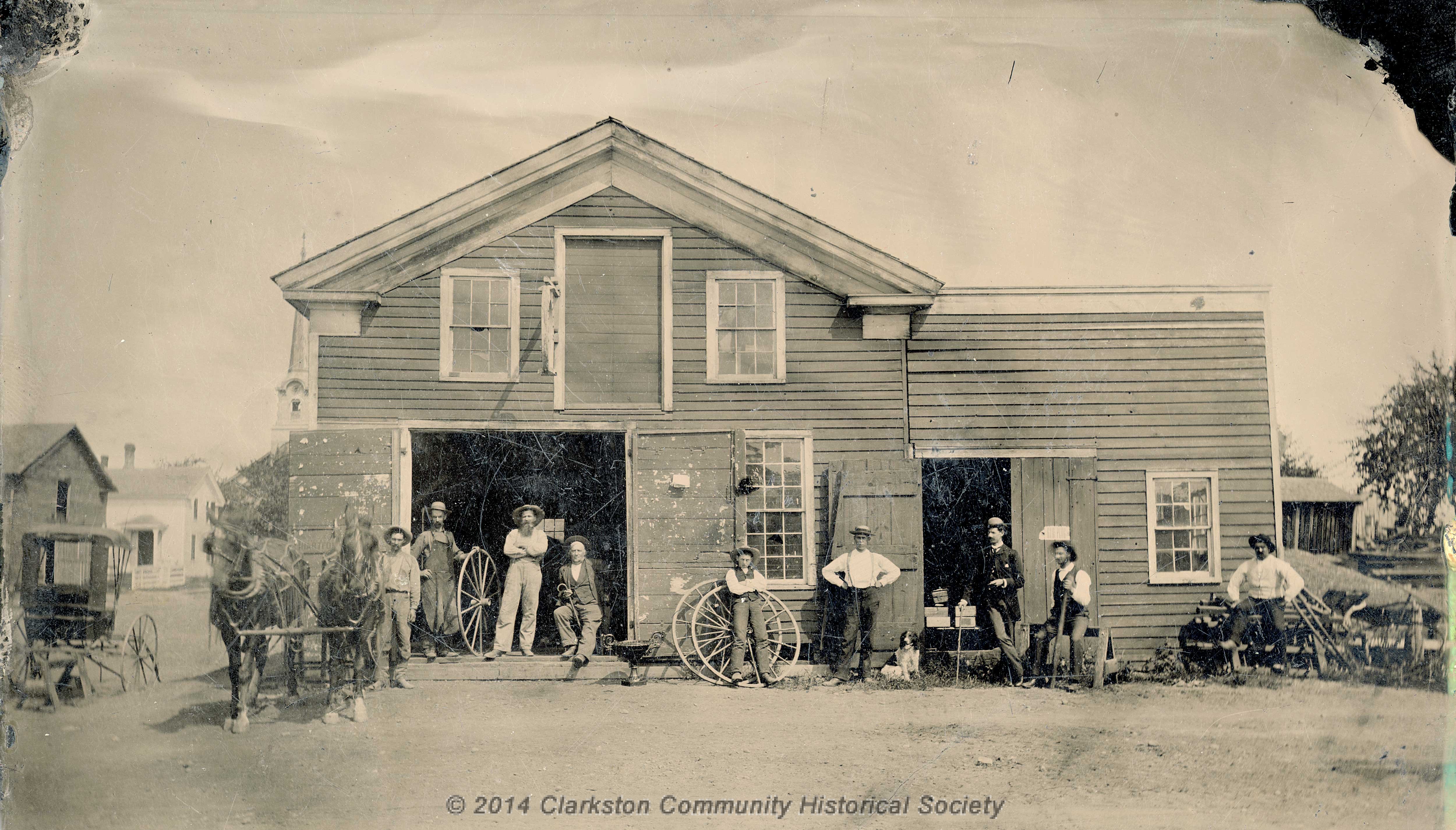This is a black-and-white photograph with a bronze tint, depicting an old wooden building that looks like a barn or a farmstead. At the bottom of the image, it says "© 2014 Clarkston Community Historical Society." In the foreground, eight people, including men and children, are posing for the camera, all dressed in old-time clothing such as overalls, long pants, white shirts, and sun hats. Some of them appear to be holding tools or parts of a wheel. To the left of the building, there are horses and a carriage, and several other buildings, including a white house and a grey house, are visible in the background along with a few trees. The upper left and right corners of the photograph have black, smokey areas, indicating some degradation of the image over time.